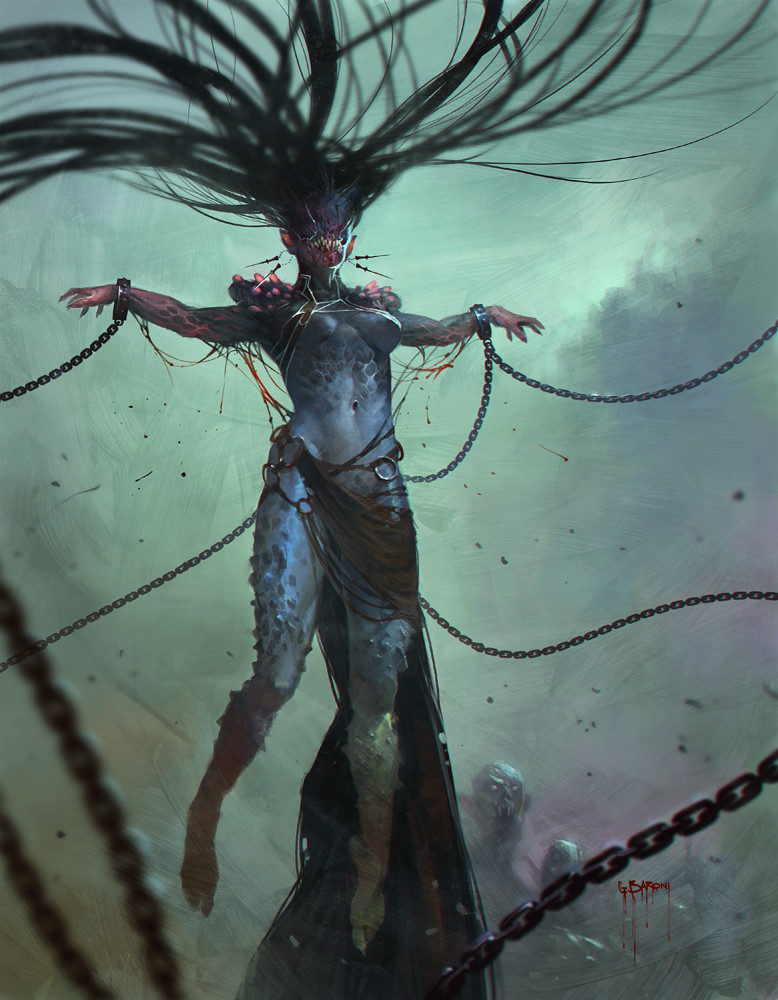The artwork depicts a haunting underwater scene featuring a woman with chains binding her wrists and waist. She is suspended with her arms raised, evoking a crucifixion pose. Her face is obscured by voluminous strands of hair that stretch across the entire top of the painting. The murky green water envelops her, revealing a wooden post or tree to which she is chained. Her skin takes on a purplish-blue hue, contrasting with her tan legs. Below her, a ghoulish figure with green eyes and exposed teeth lurks, adding to the eerie atmosphere. The bottom right corner of the painting carries a signature, possibly written in blood, that reads "G Baron." The nightmarish, demon-like transformation of the central figure, with sharp teeth and monstrous features, hints at a comic book or superhero origin.